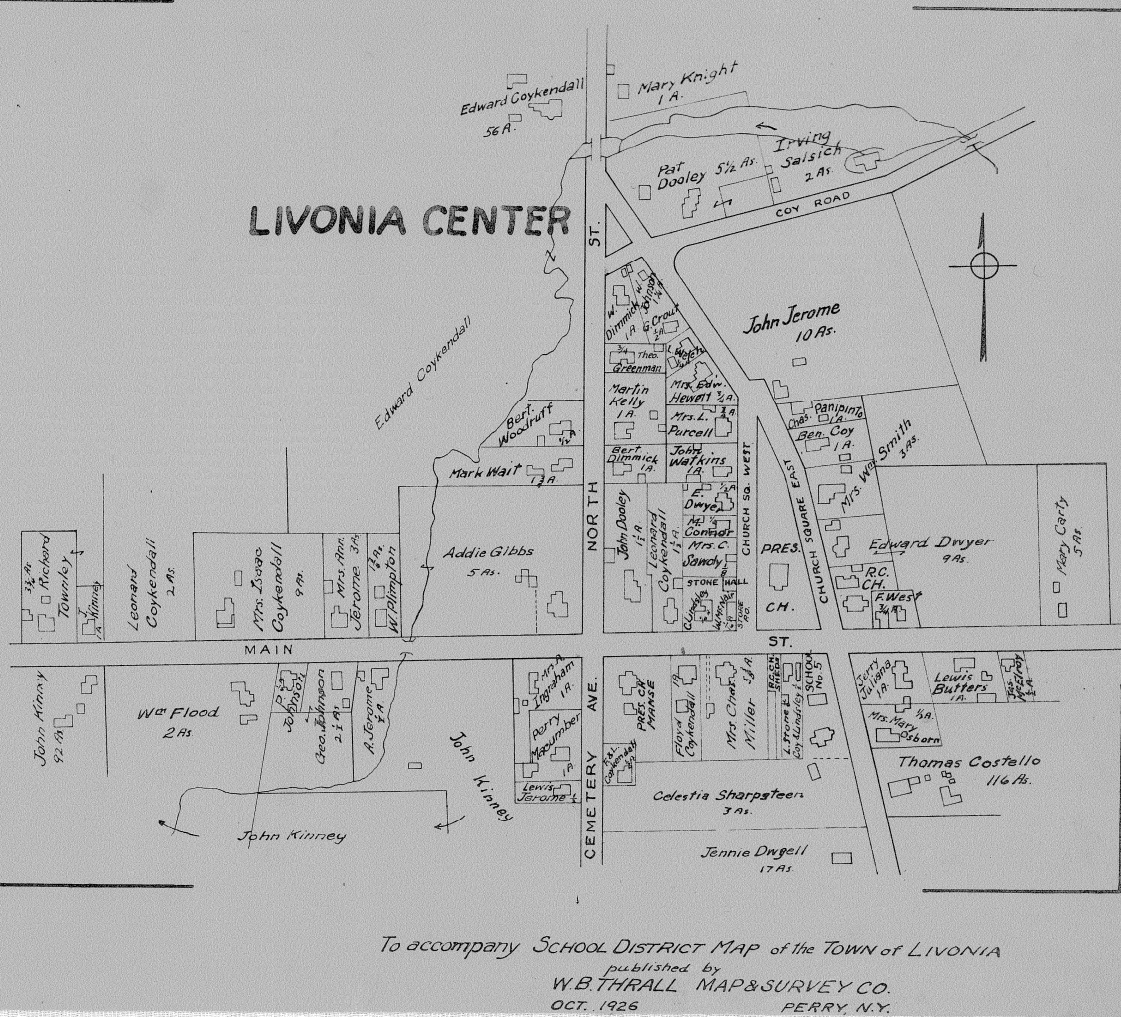The image is a meticulously hand-drawn map in black ink on gray paper, titled "Livonia Center," depicting the central area of the town of Livonia. The map is detailed with numerous streets including Main Street, North Street, and Cemetery Avenue, and it features various plots of land, each labeled with the names of their respective owners such as Celestria Sharpsteers, Jenny Dwigel, Thomas Costello, Lewis Butters, Edward Coquendale, and John Jerome among others. Additionally, notable landmarks like churches and public squares are identified. At the bottom of the map, a heading reads "To accompany school district map of the town of Livonia," and it was published by W.B. Thrall Map and Survey Corp. in October 1926 in Perry, New York. The overall depiction is straightforward and captures the layout and ownership details of Livonia Center in a clear and organized manner.